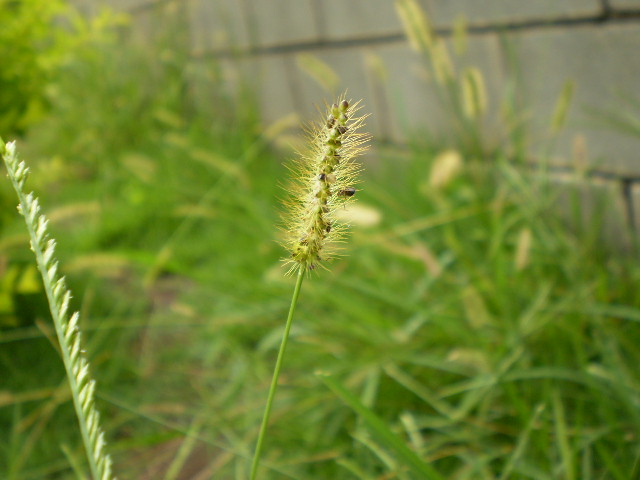The image is a slightly rectangular, landscape-format photograph, taken outdoors. It features a close-up of a piece of greenery, possibly a weed or plant, growing from the center bottom of the picture. The plant has a narrow, green stem that is sharply in focus and extends upwards. At the top of this stem, there is an inch-long, bumpy, caterpillar-like bloom, covered with greenish-yellow hairs or filaments. To the left, there is another stem or blade of grass, also in sharp focus, with a similarly rough texture. The background is blurred and consists of more greenery and tall grass, indicating it's likely taken during spring. You can also see a section of a brick or concrete gray block wall in the upper right corner, which adds a rigid texture against the natural elements. There is a suggestion of an insect hovering near the bloom, potentially feeding on the nectar. Overall, the emphasis is on the detailed structure and texture of these two stems in the foreground, set against a softly blurred natural and man-made background.